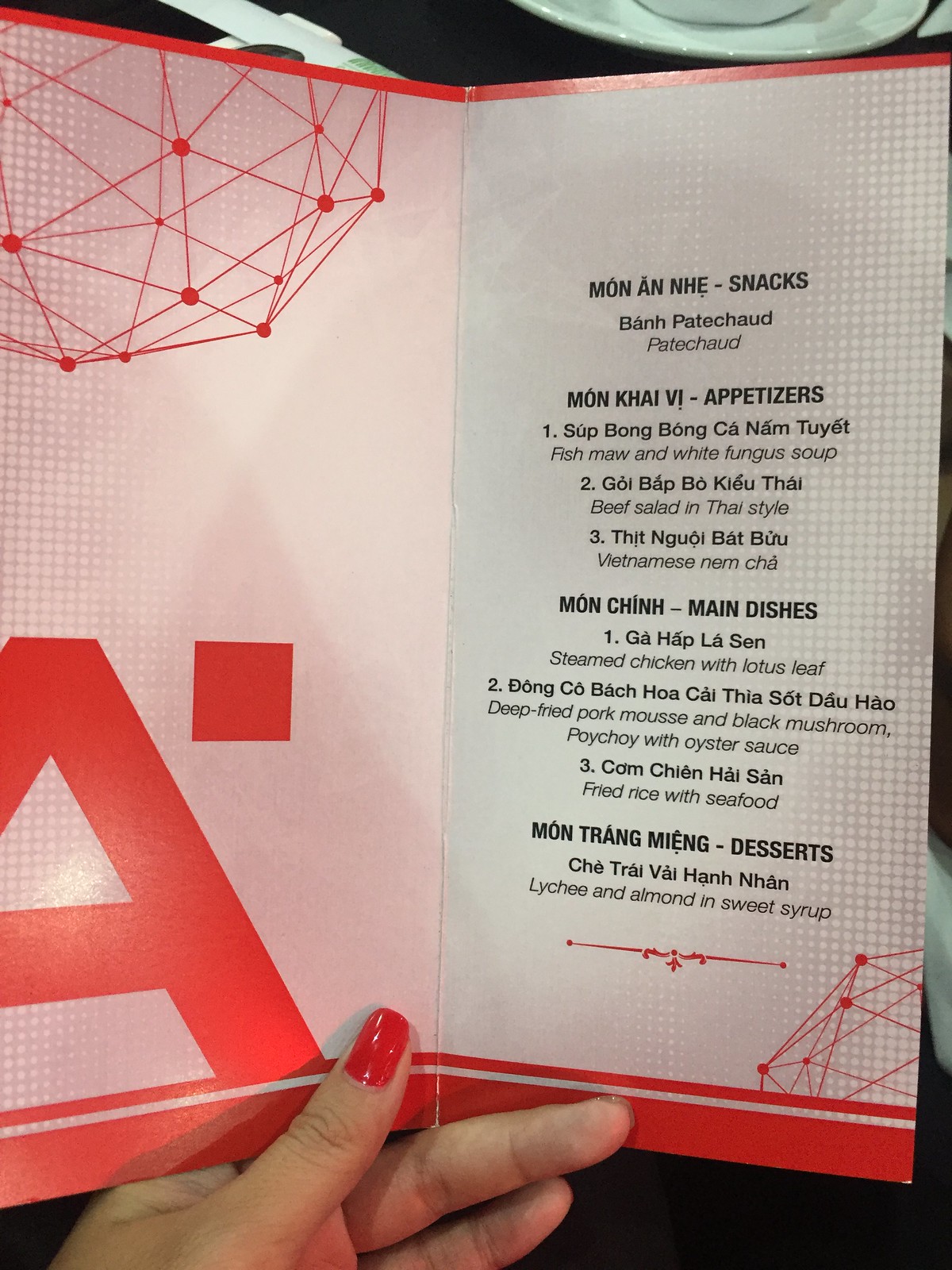In the photograph, a female hand with long, red-polished fingernails firmly holds a menu. The menu, made from a sturdy cardboard material, is presented in both Vietnamese and English languages. The upper left corner of the menu features an intricate geodesic dome line drawing, while the lower portion showcases a bold, red block letter "A". The background design consists of a pinkish-red grid that fades towards the center against a white backdrop.

The menu item list includes various sections such as snacks and appetizers. Under appetizers, some of the highlighted dishes are Fish Maw and White Fungus Soup, Beef Salad in Thai Style, and Vietnamese Nem Cha. The main courses listed include Steamed Chicken with Lotus Leaf, Deep-Fried Pork Mousse with Black Mushrooms, Khoi Choy with Oyster Sauce, and Fried Rice with Seafood. For dessert, options like Lychee and Almond in Sweet Syrup are available.

The menu is visually striking and thoughtfully organized, with a harmonious color scheme that complements the red nail polish of the hand holding it, creating a cohesive and aesthetically pleasing image.